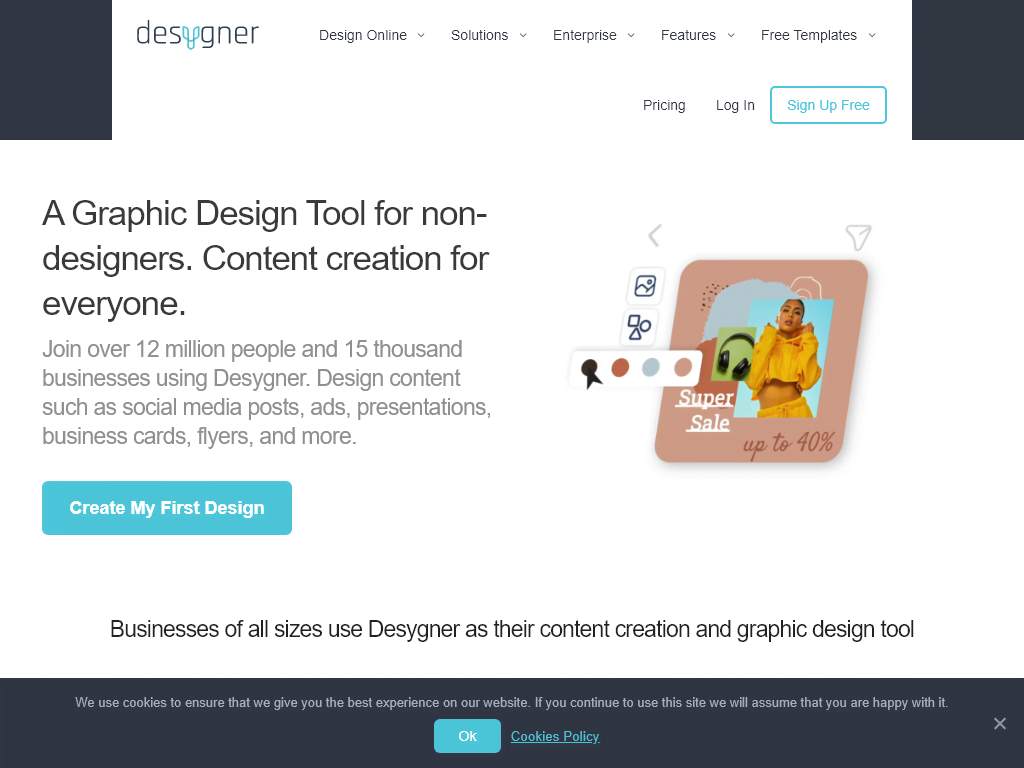The image showcases a website's homepage with a polished interface. In the top left and top right corners, there are various menu items labeled "Design Online Solutions," "Enterprise Features," "Free Templates," "Pricing," and "Login." The site prominently features the word "designer," stylized as "disYGNERS" to emphasize the creative twist.

Central to the page is a bold headline that reads, "Graphic Design Tool for Non-Designers," with a subheading that touts the benefits: "Content Creation for Everyone. Join Over 12 Million People and 15,000 Businesses Using Design Concepts and Social Media Posts, Ads, Presentations, Business Cards, Flyers." Below this, there is a call-to-action button reading, "Create My First Design."

To the right of the central content, another section includes the word "Lotto" and a photo featuring a black circle, red circle, gray circle, and brown circle, with the text "SuperSell." This section seems to highlight different designers specializing in content creation and graphic design.

At the bottom, a cookie consent message states, "We use cookies to ensure that we give you the best experience on our website. If you continue to use this site, we will assume that you are happy with it." 

Overall, the website appears to be a comprehensive tool for graphic design, aimed at both novice and experienced users, with a variety of features to enhance content creation.